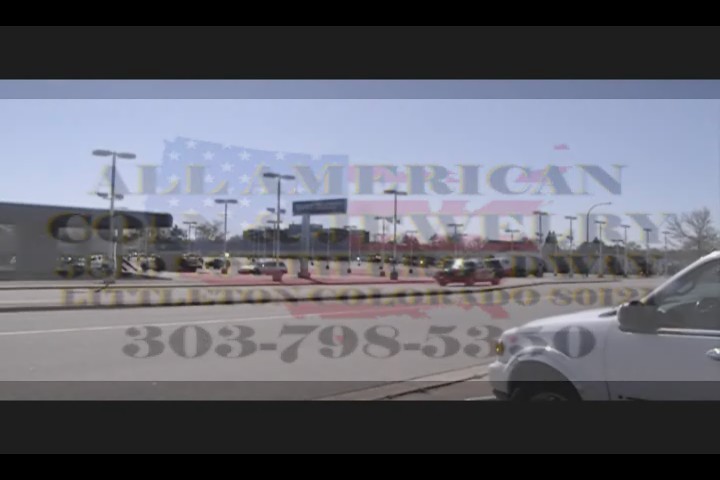The image appears to be a still frame taken from a televised video advert, presenting a somewhat grainy widescreen color image bordered by thick black horizontal lines. These lines suggest an older television format. The screen is overlaid with semi-transparent text, which is difficult to read through but displays crucial advertising information. The prominent text at the top reads "All-American" in dark grey with a yellowish outline, accompanied by a faded American flag in the background. Below that, although partially obscured, the text appears to mention "coin" and a likely "jewelry" store. Another line clearly states "Littleton, Colorado," followed by a contact number, 303-798-5330.

The background captures an exterior view of an American strip mall, featuring a parking lot populated with street lights and various parked cars, including a white car to the right and a possibly black-and-white police car on the street. The scene looks onto a busy street with a central road divider. The setting suggests it could be the advertisement's subject location, emphasizing the coin and jewelry store referenced in the text.